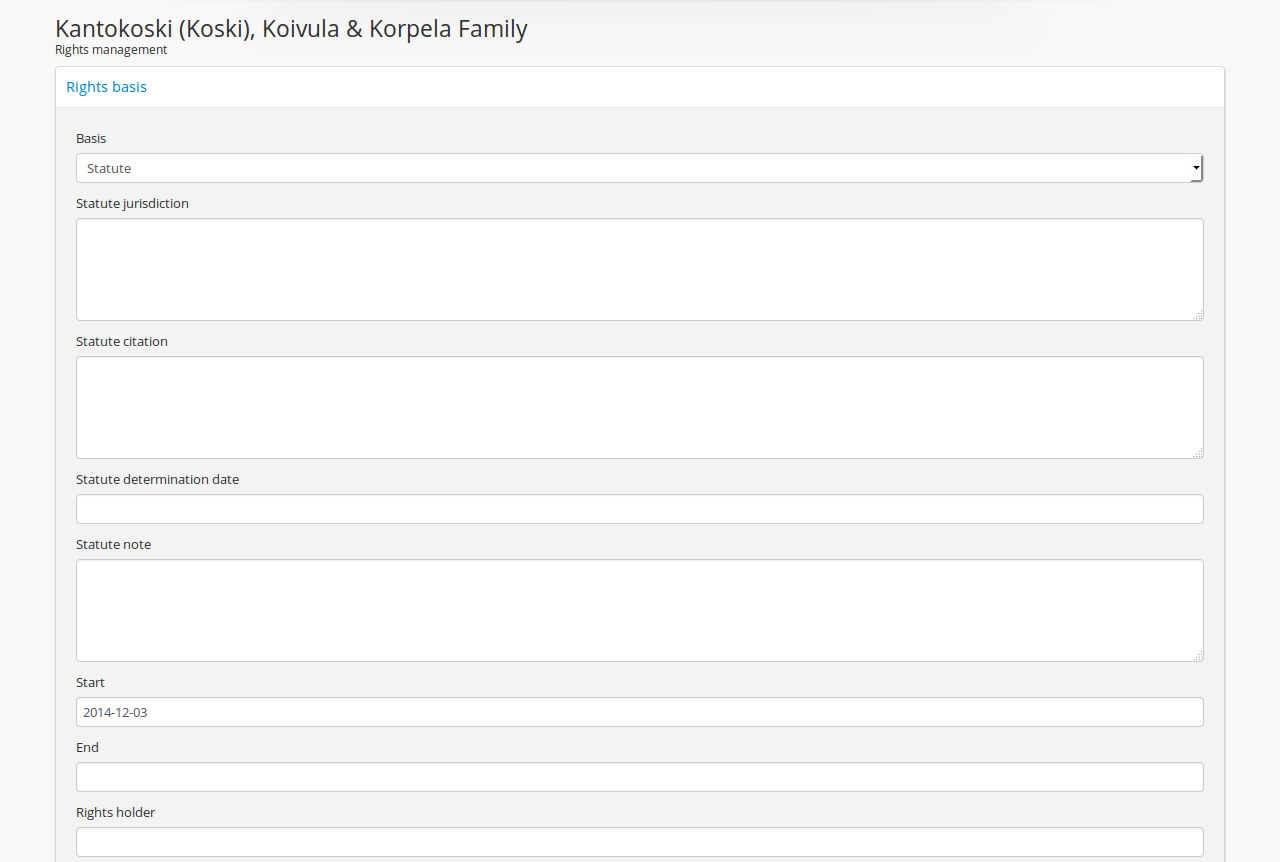This detailed caption describes an image of a specific window titled "Kanto Koshi Koshi Koivula and Korpella Family," displayed prominently at the top left corner. Directly underneath this title, "Rights Management" is written. Within the window, there is a primary box labeled "Rights Basis" at its top left side. Inside this larger box are several smaller sections:

1. **Basis:** A drop-down menu is available here, with "Statute" currently selected.
2. **Statute Jurisdiction:** This section contains a small window for inputting the relevant jurisdiction.
3. **Statute Citation:** Similar to the previous section, it provides space to write the statute citation.
4. **Statute Determinant on Date:** There is a white bar to enter the specific determinant date.
5. **Statutory Note:** This area also follows the same input format.
6. **Start Date:** The start date is filled in as "2014, December 3".
7. **End Date:** This field is left empty.
8. **Rights Holder:** This section is also left empty.

These fields are clearly designated for users to input various specific details regarding rights management.